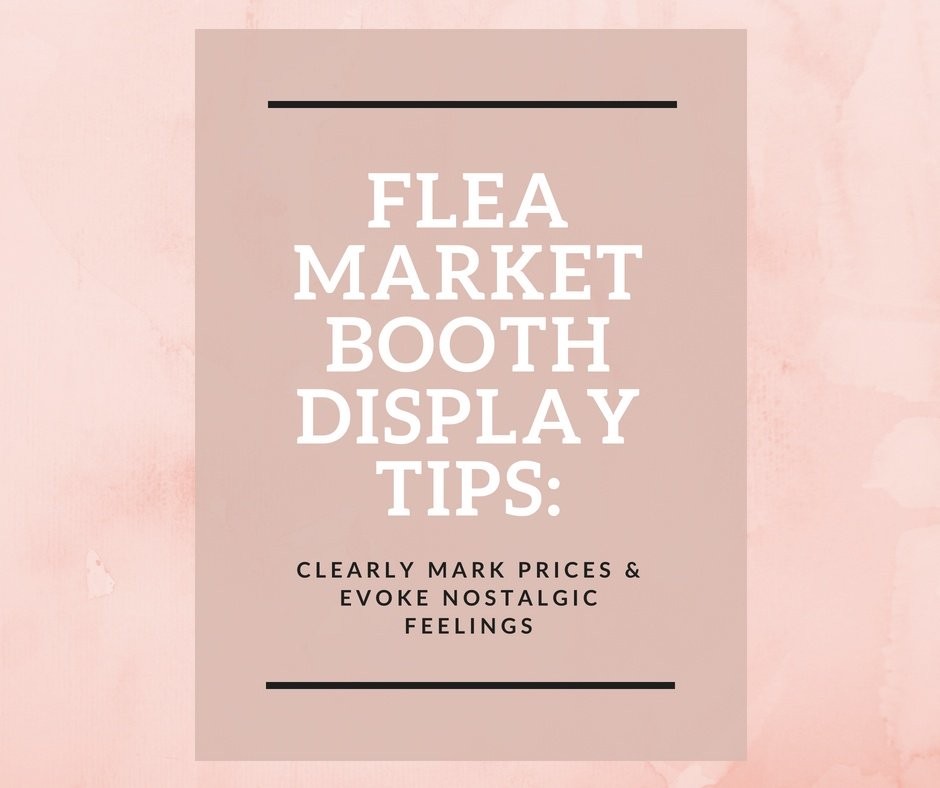The image features a square graphic set against a light pink background with subtle watercolor splotches. In the center, there's a slightly darker purple rectangle that occupies most of the image's height. This central rectangle is bordered by black horizontal rules near the top and bottom. The main text within the rectangle is in large white font and reads, "Flea Market Booth Display Tips," with each word on a separate line and center-aligned. Below this main heading, in smaller black font, are the tips: "Clearly mark prices and evoke nostalgic feelings." The graphic serves as an instructional guide for creating effective flea market booth displays.